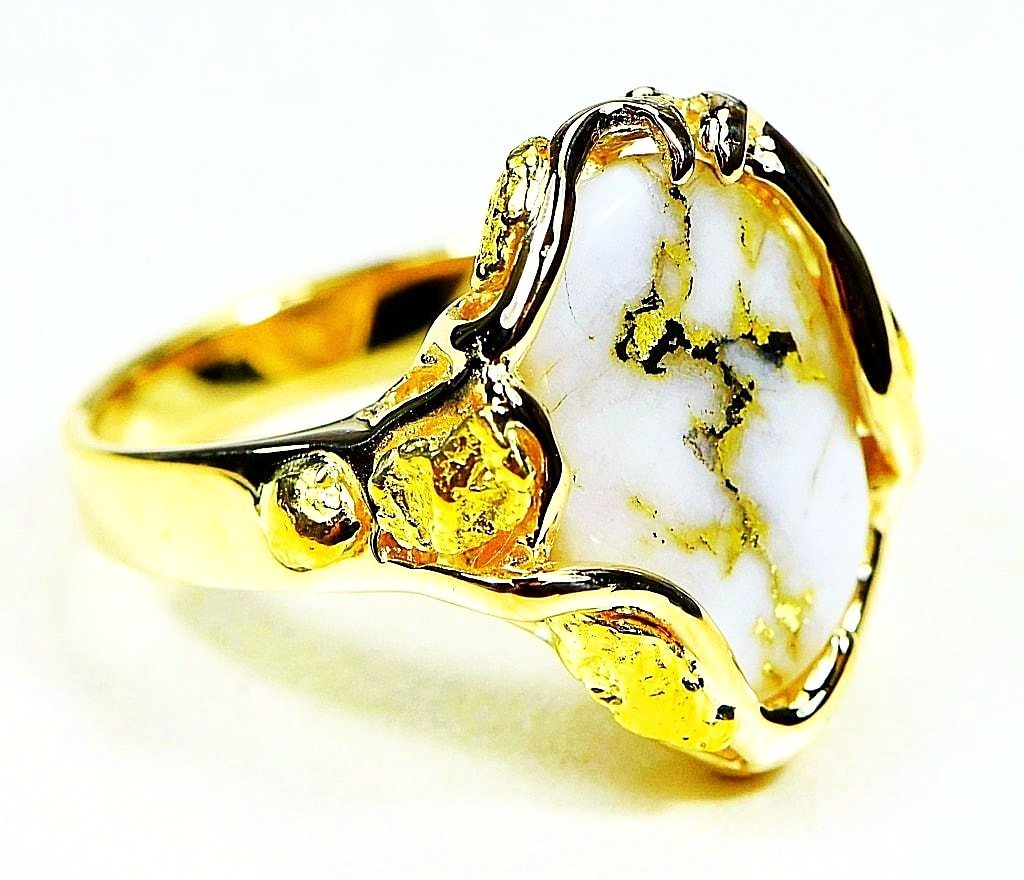The image features a close-up of a highly reflective gold ring with a unique gemstone set at the top. The stone is predominantly white with intricate patterns of yellow and black running through it, creating a striking visual effect. There are hints of burnt orange near the stone's edge, adding to its complexity. The ring is positioned at a slight tilt, with the gemstone centered but slightly to the right, while the band extends to the left in the background, casting a subtle shadow on the white, slightly blurry surface beneath. The ring does not appear symmetrical and has a rough, uneven design, particularly noticeable in the gold setting holding the gemstone. There is no accompanying text, suggesting the focus is purely on the visual details of the ring. The image is brightly lit, causing significant glare that accentuates the gold and makes some details challenging to discern. The overall color palette is limited to gold, white, black, and touches of burnt orange, all highlighted against the nondescript white background.